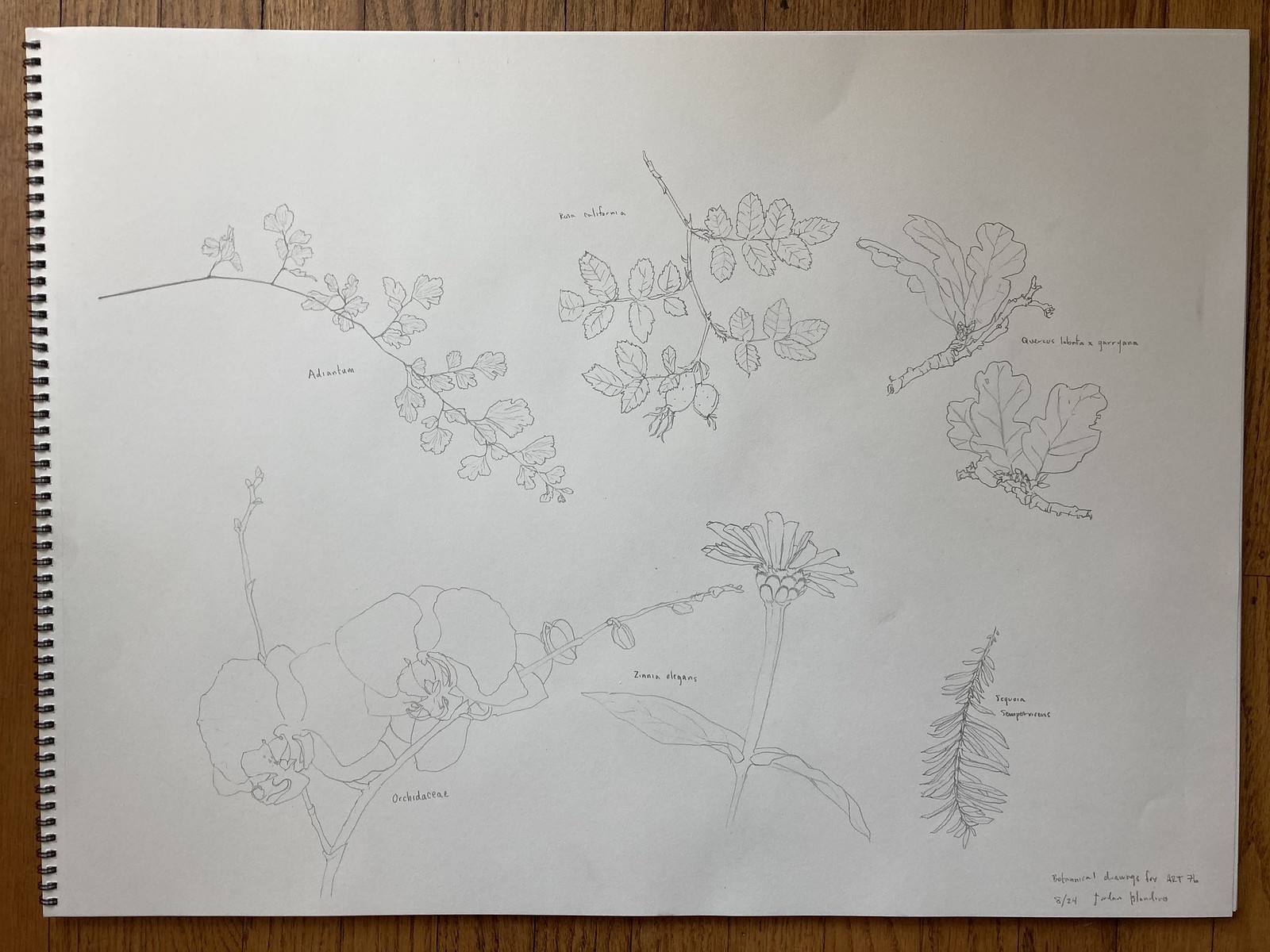The image features a detailed sketch of various plants on a large, white, spiral-bound notebook resting on a dark brown wooden table. The white paper, which appears light gray in places, occupies 90% of the image and has a series of black holes from the spiral binding on its left-hand side. There are six distinct hand-drawn sketches of plants, primarily vines with leaves, although one flower is depicted in the bottom center with a leaf to its right. These illustrations appear to be scientific drawings, each labeled with extremely small text. The top three sketches resemble trees with foliage, while the bottom three include flowers and what looks like part of the fronds of a pine tree. All drawings are executed in black pencil and partially colored in. The artist has signed and dated the bottom right corner of the page.